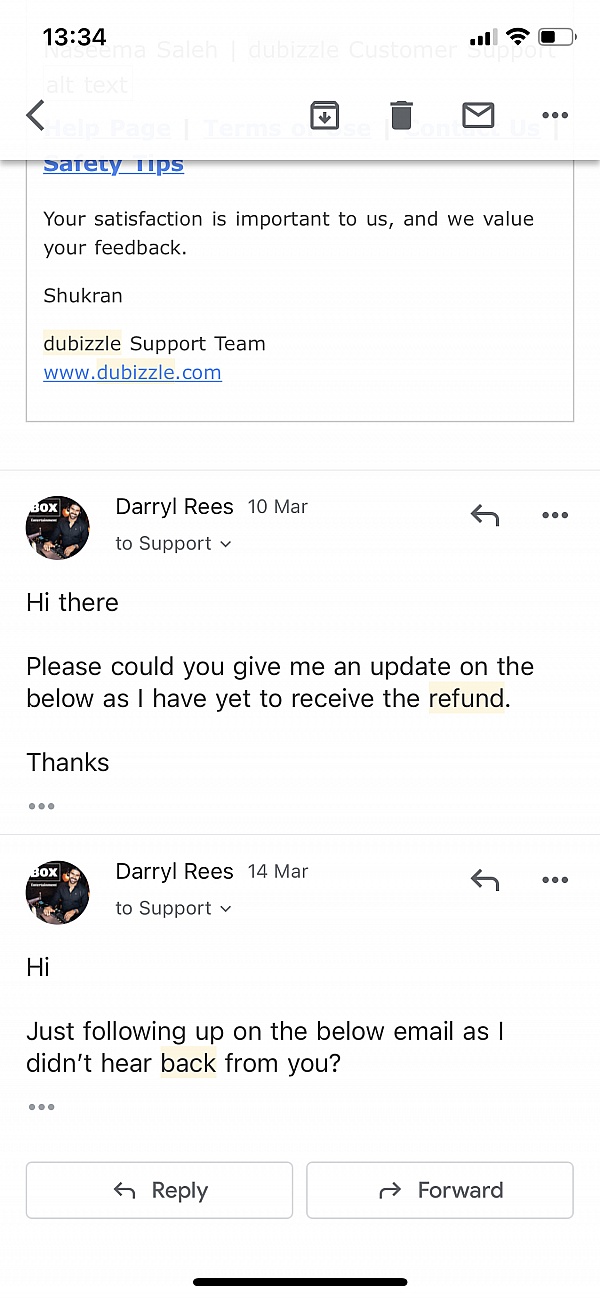### Detailed Caption for Image:

The image is a screenshot of an email chain taken from a smartphone. At the top of the screen, the status bar displays the time as 13:34, with three out of four bars indicating cellular signal strength, full Wi-Fi connectivity, and the battery at around 40%. Just below the status bar, there are several interface buttons: a back button, a download button, a trash icon, a reply button, and a hamburger menu.

Continuing down the screen, a blue hyperlink labeled "safety tips" is displayed. Below it, there's a statement in black text that reads: "Your satisfaction is important to us and we value your feedback." This message is signed off by "Sucron, Dubizzle support team," with another hyperlink, "dubizzle.com," placed underneath.

Further down, there's a profile picture of a man dressed in black, seated at what appears to be either a piano or a guitar, set against a black background. The name "Daryl Reese" accompanies the photo, followed by the date "10 March", and the recipient "to support."

In his message, Daryl Reese writes: "Hi there, please could you give me an update on the below as I have yet to receive the refund, thanks." This section also contains a hamburger menu to the right of Daryl’s name.

A follow-up email from the same individual, Daryl Reese, is timestamped "14 March", also sent "to support". In this message, he writes: "Hi, just following up on the below email as I didn't hear back from you?" A hamburger menu icon is present here as well.

At the bottom of the email thread, there is an option to "reply and forward". Notably, the words "refund" and "bag" are highlighted with a yellow background throughout the email chain.